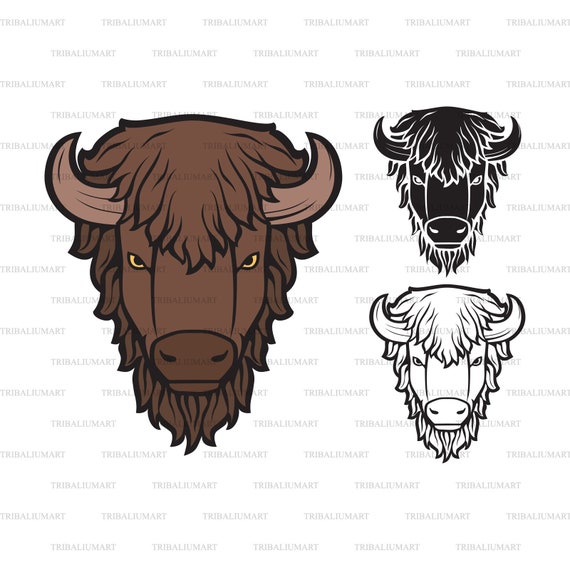The image is a detailed vector art logo design showcasing the head of a horned animal, possibly a buffalo or bison. There are three versions of the head, each in different stages of design, set against a white background. The main, most detailed image on the left features a brown buffalo head with yellow eyes and lighter brown horns, accented with shadows and gradients for a realistic effect. To the right are two smaller, less-detailed versions: one in black and white line art, and the other an inverted version with black outlines on white. The background of the image is obscured by repeated text that reads "Tribal mart" or "Tribali mart" in plain, duplicated fonts. This design showcases different stages and styles of the logo, illustrating its versatility for potential use in various applications such as clothing or accessories.